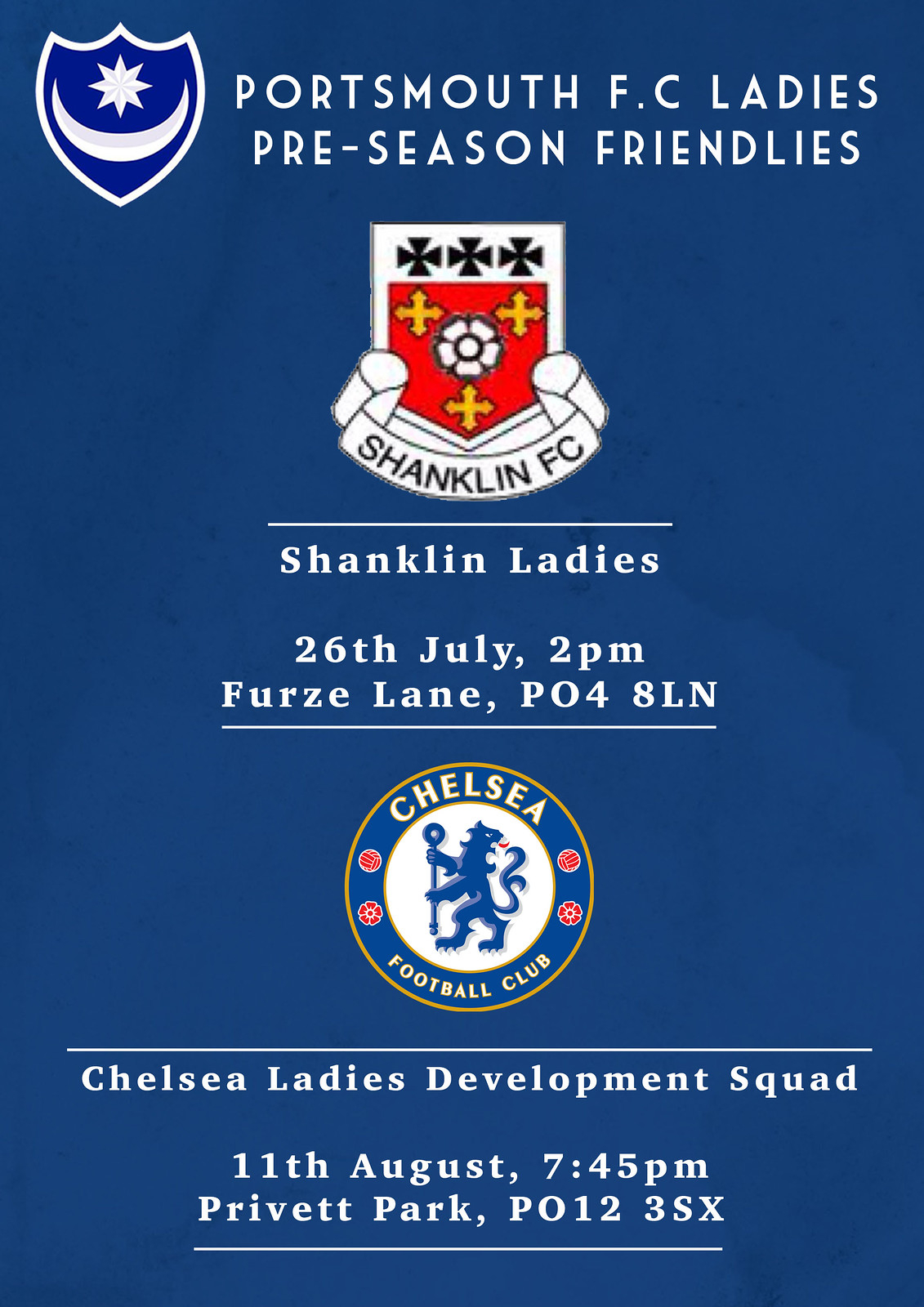This poster features a dark blue background with white text announcing Portsmouth FC Ladies' pre-season friendlies. Positioned in the top left is the Portsmouth FC logo, depicted as a white shield containing a starburst and a crescent moon. Centrally placed but slightly towards the top is the Shanklin FC logo, which is adorned in red, gold, white, and black, including crosses and a flower motif, with a white ribbon below it displaying "Shanklin FC". Below this is the detailed information: "Shanklin Ladies 26 July 2 p.m. Ferds Lane PO48LN." Further down is the Chelsea Football Club logo, a blue and white circular emblem with additional gold and red accents. The text beneath reads: "Chelsea Ladies Development Squad 11th August 7:45 p.m. Privet Park PO12 3SX." White lines separate each section, emphasizing the details and making the advertisement clear and organized.